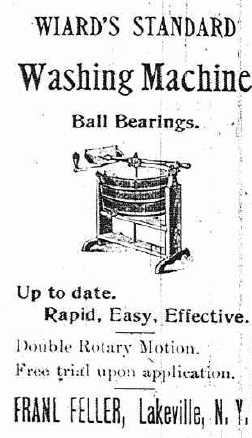This is an image of a very old newspaper or magazine advertisement for the "Weyard's Standard Washing Machine." The advertisement features a white background with black text, some of which is faded and shows signs of bleed-through from the printing process. At the top, the ad prominently displays "Weyard's Standard" in bold font, followed by "Washing Machine" in slightly larger mixed upper and lower case font. Below this, in smaller font, it states "ball bearings."

In the center of the image, there is an illustration of an old-fashioned washing machine. The drawing depicts a wood barrel on a platform with a handle on top, which likely enables a double rotary motion for washing. The contraption is stabilized by wooden pieces. 

Below the picture, the advertisement touts the machine's features with the text: "up-to-date, rapid, easy, effective, double rotary motion, free trial upon application." At the very bottom, it reads "Franl Feller, Lakeville, New York," although the name appears inaccurately written in the third interpretation as "Fresnel Feller."

The overall text-based design and black-and-white color scheme give the ad a very antiquated appearance, suggesting it could plausibly be from a much earlier time period.